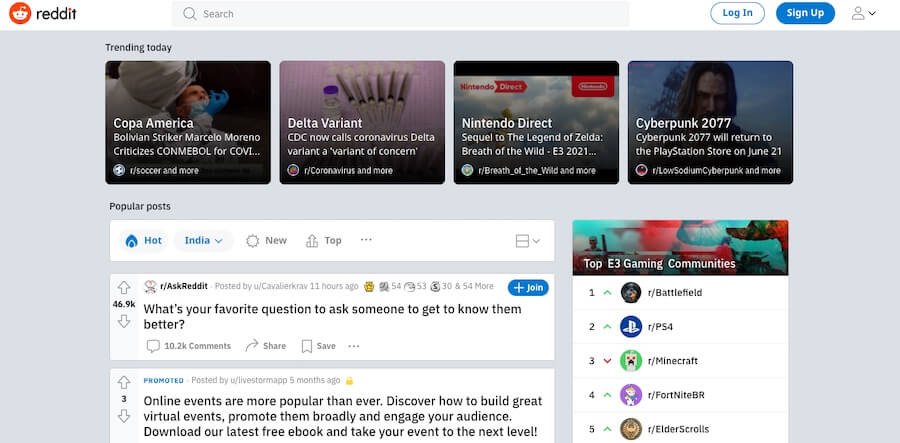The image depicts a Reddit webpage. At the top left corner, there is the Reddit logo followed by the word "reddit" in black text. Next to this is a gray search bar. To the right of the search bar, there are two buttons: a button to log in and a bright blue button to sign up. Following these, there is an icon representing people.

Directly below this header area is a horizontal rectangular box with a light blue background. At the top of this box, there is a heading that reads "Trending Today." Below this heading, there are several topics that are popular for the day. The topics are each accompanied by an image and are listed from left to right: "Copa America," "Delta Variant," "Nintendo Direct," and "Cyberpunk 2077," with the corresponding subreddits mentioned below each topic.

Underneath this section, in small black text, is the label "Popular Posts." Directly below this, there is a highlighted post from the "hot" category in the AskReddit subreddit. The post features the question, "What's your favorite question to ask someone to get to know them better?" and has received 46.9 thousand likes.